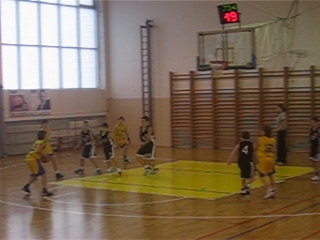In this tiny photograph of a youth basketball game, the focus is on the action around half court. The gym's key, including the free throw line, is brightly colored in yellow, standing out prominently on the court. Two teams are in play: one dressed in yellow uniforms and the other in either black or white. Near the hoop, a referee is clearly visible, overseeing the game. Directly above the hoop, a digital timer displays "49" in red digits, indicating the time left. To the left side of the court, large, multi-paned windows flood the gym with daylight, emphasizing that the game is taking place during daytime.